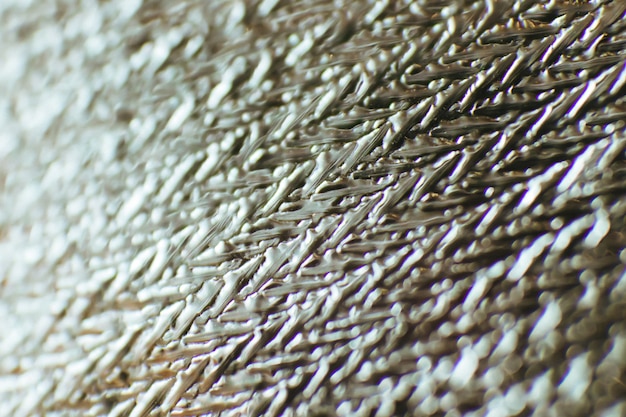This rectangular photograph is a highly detailed, close-up image of a woven textile featuring a pattern of V-shaped chevrons arranged in diagonal rows. The fabric, which could potentially be yarn, braid, or embroidery, showcases shades of dark gray, black, and silver, with a metallic sheen that is most pronounced under natural or studio light. This reflective quality is particularly noticeable in the upper left corner where the light intensifies the silver tones to the point of appearing almost white, obscuring the pattern. The ridges, or V-shaped chevrons, extend from the bottom right to the upper left corner of the image, becoming clearer and more defined toward the center while appearing blurred at both ends. This blur creates an intriguing gradient effect, enhancing the texture and depth of the fabric. The intricate pattern and sheen suggest an artificial rather than handmade creation, giving the piece an aesthetic that echoes the look of seaweed or metallic tones, adding to its visual appeal.